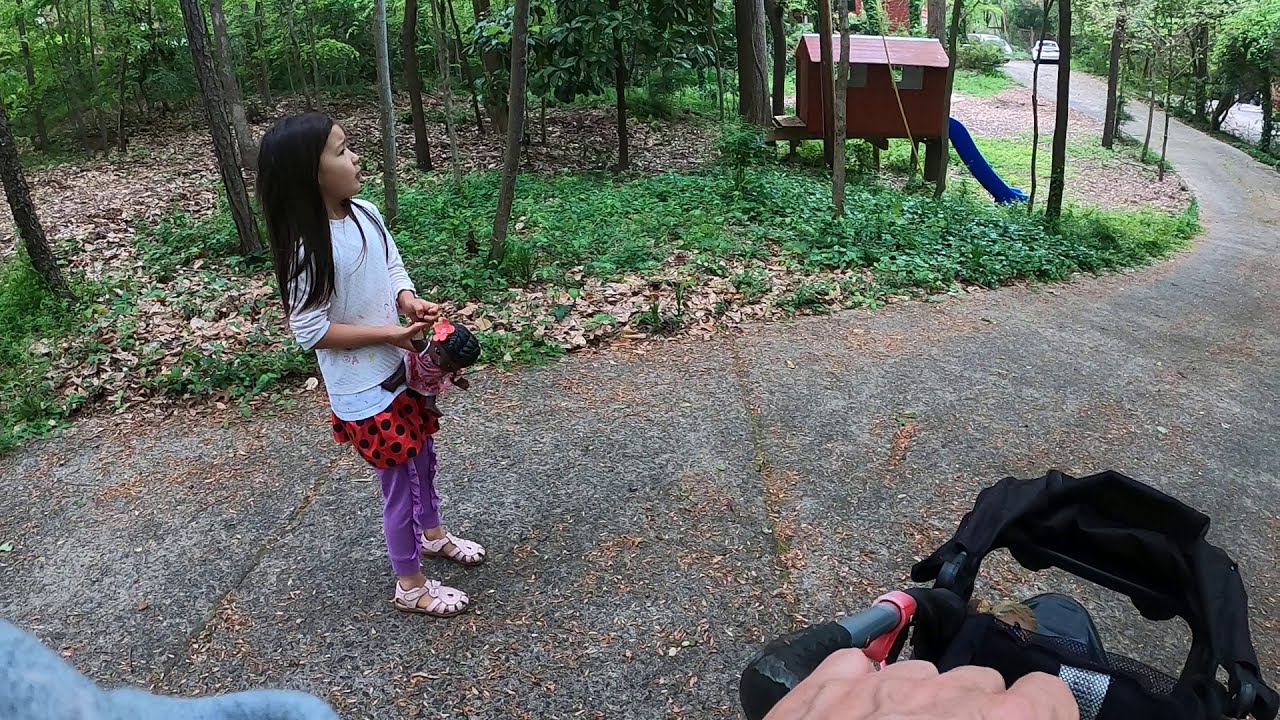In this charming full-color outdoor photograph, the scene captures a picturesque nature setting. The background features a variety of trees with scattered fallen leaves, dense bushes, and a small treehouse perched on stilts, complete with a blue slide. Off in the distance, the back of a white car and a roadway are visible. The photograph is taken from the perspective of an adult pushing a baby stroller, whose hand is seen in the lower right-hand corner. Peeking adorably from the stroller is the top of a baby's head.

Dominantly placed to the left of the stroller, a young girl with beautiful long black hair draws attention. She is joyfully dressed in a mix of a white shirt layered under a ladybug-patterned skirt, purple pants, and white sandals, though one account describes them as pink. She is carrying a doll that shares her black hair, looking off to the right, seemingly absorbed in her own world. The vibrant details of her attire and the surrounding lush greenery come together to create an endearing and lively snapshot of a simple, yet heartwarming moment.